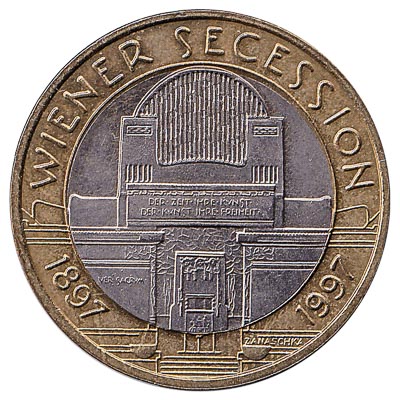The image features a coin as the central focus against a white background. The coin has a brassy, corroded-looking outer ring with an etched border and the inscription "Wiener Secession" along the top edge. The bottom edge displays the years "1897" on the left and "1997" on the right. The coin's center is raised and has a more silver or purplish tint, appearing fairly worn rather than shiny. Prominently featured in the center is a depiction of a dome-like structure, possibly part of a building, with unreadable text that appears to be in German. The building includes a door-like feature at the front, flanked by what seems to be stairs and railings.